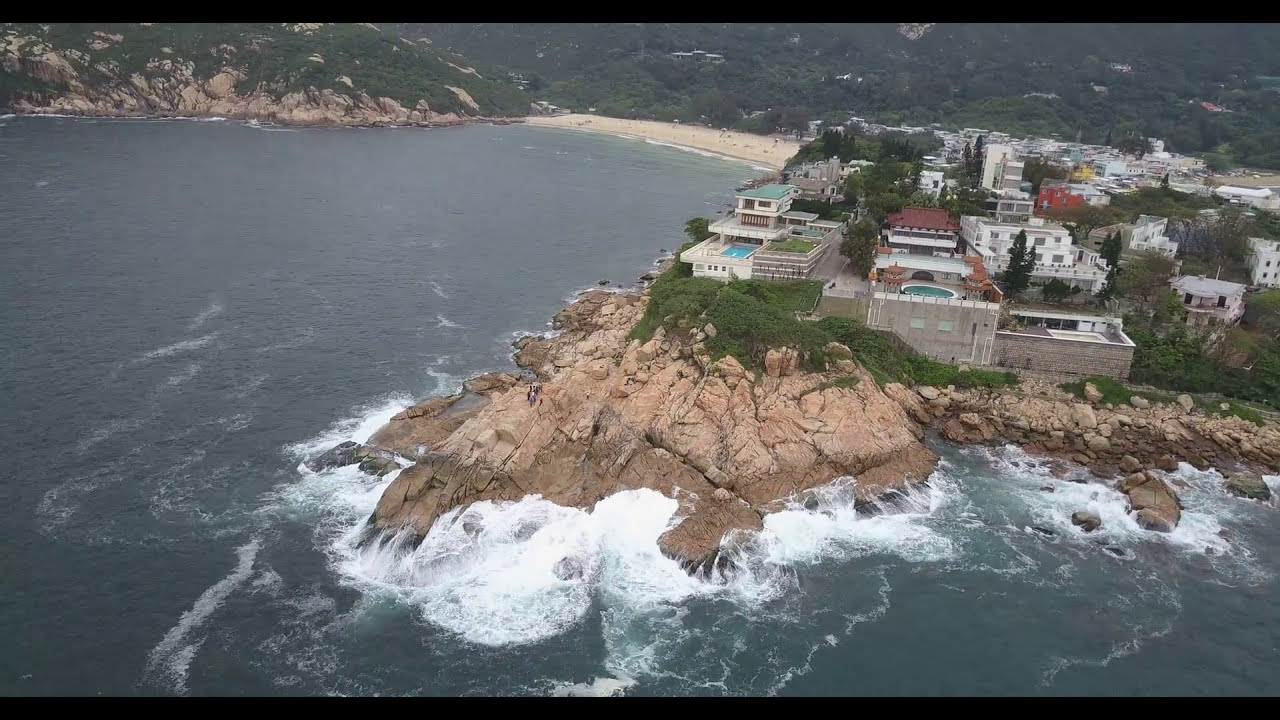This somewhat faded, full-color aerial photograph, likely taken from a drone or helicopter, captures an expansive daytime view of a coastline. In the foreground, the dark blue ocean aggressively meets a massive, brown rocky outcropping, creating frothy white waves. Upon closer inspection, one can spot tiny figures atop the rocks, adding a sense of scale to the imposing cliffs. Atop these cliffs sit very high-end, multi-million dollar homes, many constructed on cement blocks and adorned with swimming pools. Surrounding the homes is lush green foliage. In the upper center of the image, a brown, sandy beach dotted with scattered beachgoers transitions into a bay area. Beyond this, a rocky hillside covered in green trees extends across the horizon, giving way to a few more scattered houses. The photograph has a gray cast, suggesting an overcast sky, and features narrow black borders at the top and bottom.